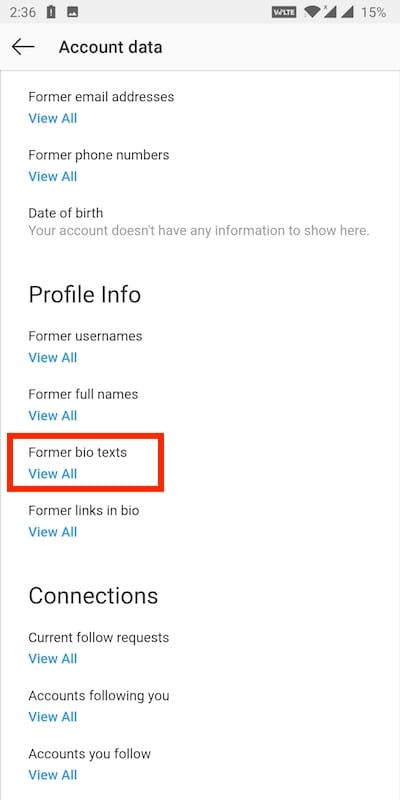This mobile screenshot displays the "Account Data" tab. At the very top, a green header with bold black letters reads "Account Data," accompanied by a left-facing arrow on the left side. Below this header, the background transitions to white.

The first section is labeled "Former Email Address," with an option to "View All" in blue immediately below it. Following that, there is a section for "Former Phone Numbers," which also includes a "View All" option. Next is the "Date of Birth" section, which contains the text, "Your account doesn't have any information to show here," in small gray letters.

A section titled "Profile Info" follows, highlighted with large black letters. This section lists "Former Usernames," "Former Full Names," and "Former Biotexts." Notably, the "Former Biotexts" section is emphasized with a red box around it. Further down, there is a section for "Former Links in Bio."

At the bottom, a segment labeled "Connections" in large black letters appears. This includes sub-sections for "Current Follow Requests," "Accounts Following You," and "Accounts You Follow."